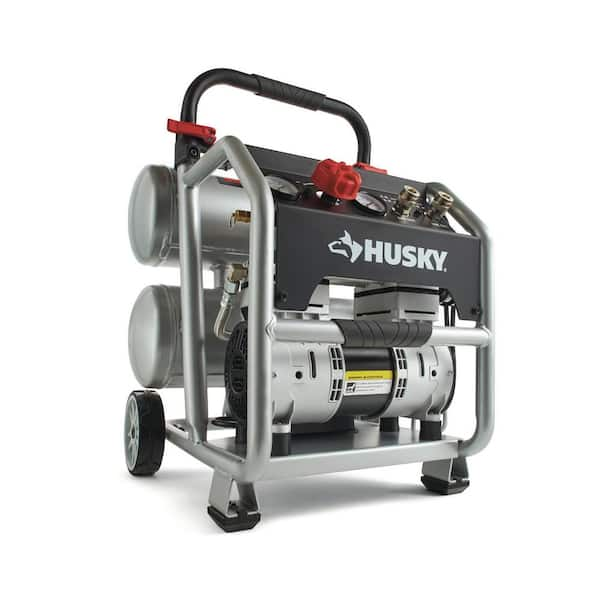The photograph features a Husky-branded electric air compressor set against a clean, white background. The compressor, identifiable by its prominent black front panel with the white Husky logo and a simplified, cartoonish husky dog's face, showcases a functional design. Central to its face are two pressure gauges resembling clock faces, along with a red knob and several silver inlets and purple tubes, indicative of its versatile utility, such as inflating tires. The machine comprises three major cylindrical components — one in the front and two in the rear. The compressor is mobile, equipped with a black handle on top and wheels at the back, allowing it to be easily maneuvered. The sturdy silver base, featuring solid front legs, ensures stability when the compressor is set down.